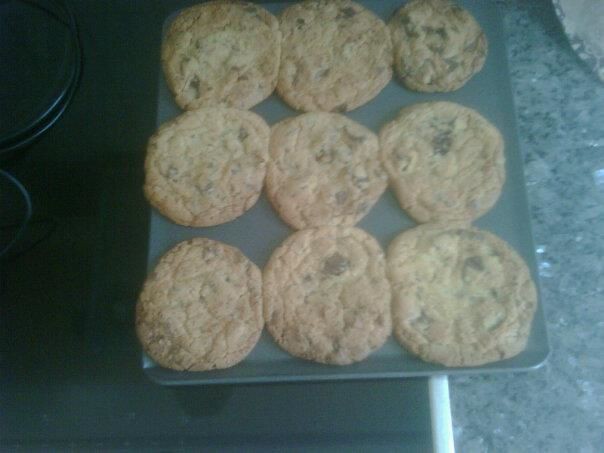The photograph captures a freshly baked batch of nine round chocolate chip cookies, arranged in three neat rows of three on a dark gray, rectangular baking pan. The cookies are a light golden brown with crispy tops, featuring small cracks and scattered with dark brown, melted chocolate chips. The perspective of the image is from above, allowing a clear view of the cookies’ flat, slightly spread shape. In the background, there is a black stovetop to the left, and to the right, a glossy gray quartz countertop with dark specks, adding a textured and polished appearance to the overall kitchen scene.